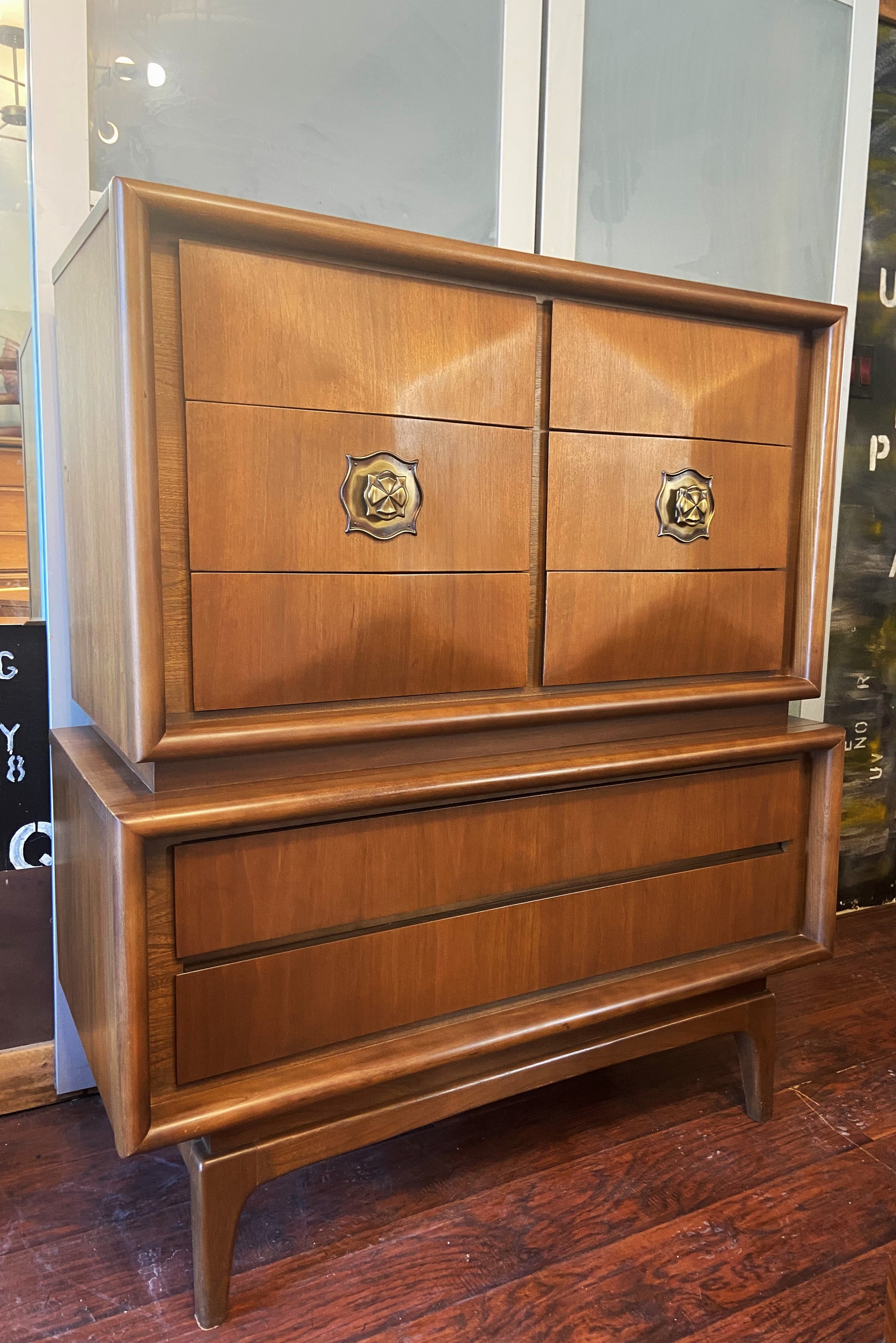The image depicts a detailed wooden hutch, standing approximately 4 feet tall, fashioned from medium to dark brown wood. The structure rests on four wooden legs, positioned on a reddish wooden floor. The hutch's base comprises one or two long, horizontal drawers. Above these drawers, the hutch transitions into a slightly inset middle section. The upper portion of the hutch features two hinged doors adorned with brass-colored clover-shaped handles situated in the center of each door, suggesting a fanciful and elegant design. The overall finish of the hutch is a medium to high gloss, enhancing its refined appearance. The piece is set against a background that includes various items and possibly frosted glass, framed by a neutral white closet with gray trim.